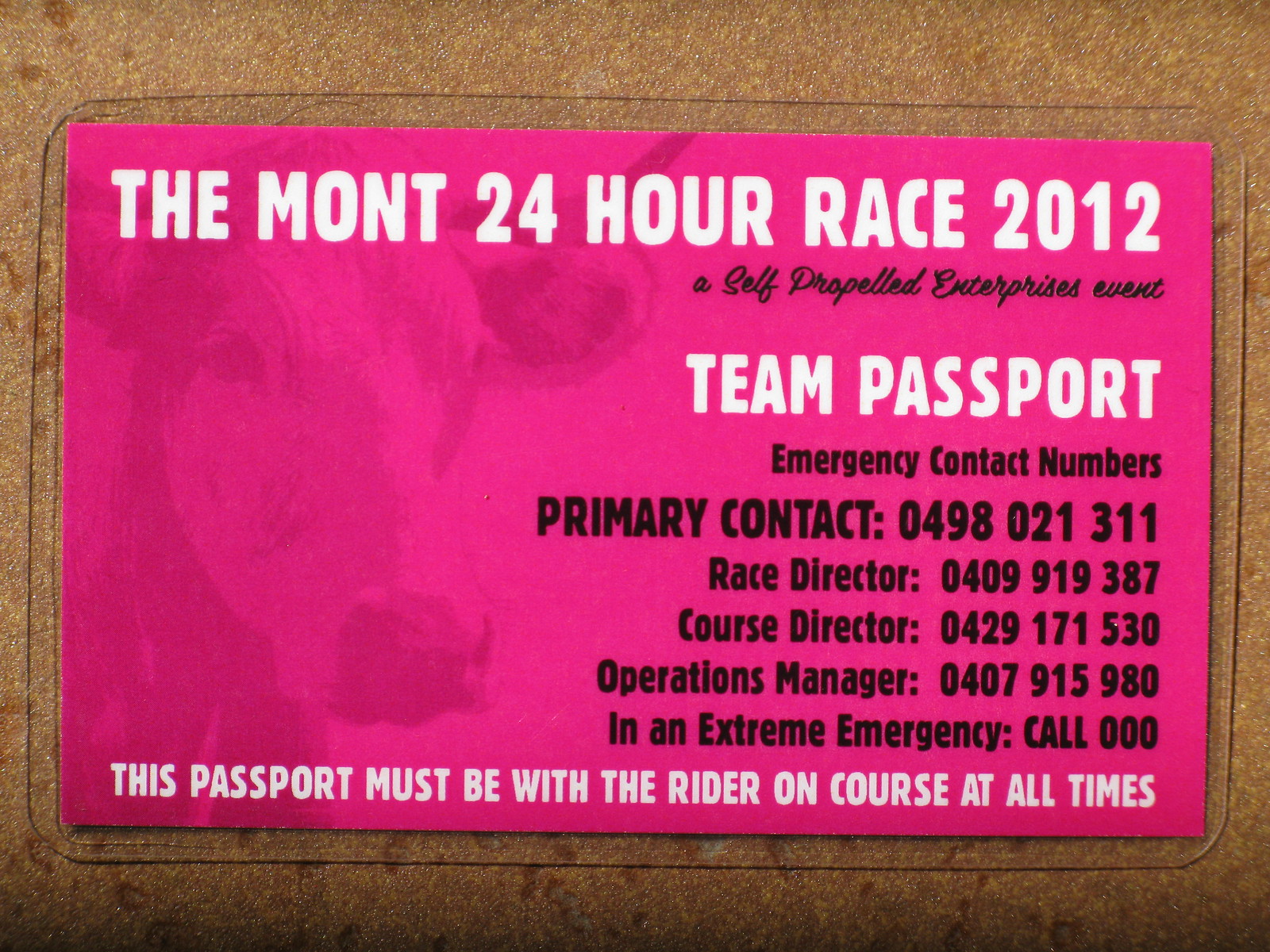The image depicts a photograph of a laminated, rectangular, pink card, laying on a beige, corkboard-like background. The card is designed as a Team Passport for The Mont 24-Hour Race 2012, a self-propelled enterprises event. Prominent at the top in large white letters is "The Mont 24-Hour Race 2012". Below this, in cursive black text, it reads "A Self-Propelled Enterprises Event". Further down in large white letters is "Team Passport". On the left side of the card is a faint drawing of a cow's face in varying shades of pink and dark gray. In black text, the card lists emergency contact numbers for various officials: Primary Contact, Race Director, Course Director, Operations Manager, and an instruction for extreme emergencies to call 000. At the very bottom, it states in white letters, "This passport must be with the rider on course at all times."